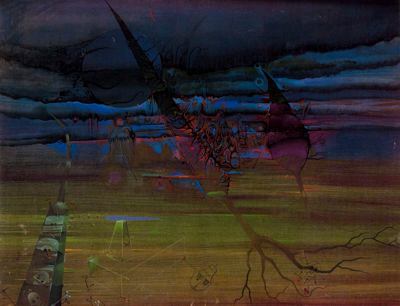In this abstract painting, the artist employs a very dark color scheme primarily featuring shades of black, navy, blue, purple, and green. The composition appears to depict a surreal landscape with indistinct forms. At the top of the painting, dark clouds made up of black and navy hues create a brooding atmosphere, with translucent gray layers overlaying black outlines that give a sense of depth and movement as they hang and blend together.

Descending towards the horizon, the scene transitions into a dark blue area, suggestive of a lake or body of water, though its abstract nature makes it ambiguous. The painting further moves into earthy tones of green and brown, creating streaks across the canvas that evoke the sense of ground or foliage.

Interspersed within the lower half of the artwork, one can discern root-like structures and possibly tree limbs, cutting through the painting at angles, depicted with black and brown lines. These elements contribute to a feeling of natural chaos and juxtaposition within the abstract environment.

Adding to the complexity, the middle section of the painting contains cone-shaped and rounded forms in black and purple, accompanied by black squiggly lines that further mystify the scene. These shapes might represent submerged or partially hidden objects, adding to the enigmatic quality of the landscape.

Overall, the painting's marble-like blend of colors transitions in an ombre effect from dark gray to light blue, deepening into purple and mauve in the center, and finally merging into sea green and soft brown below, capturing the essence of a landscape at dusk with intricate, overlapping patterns and textures.